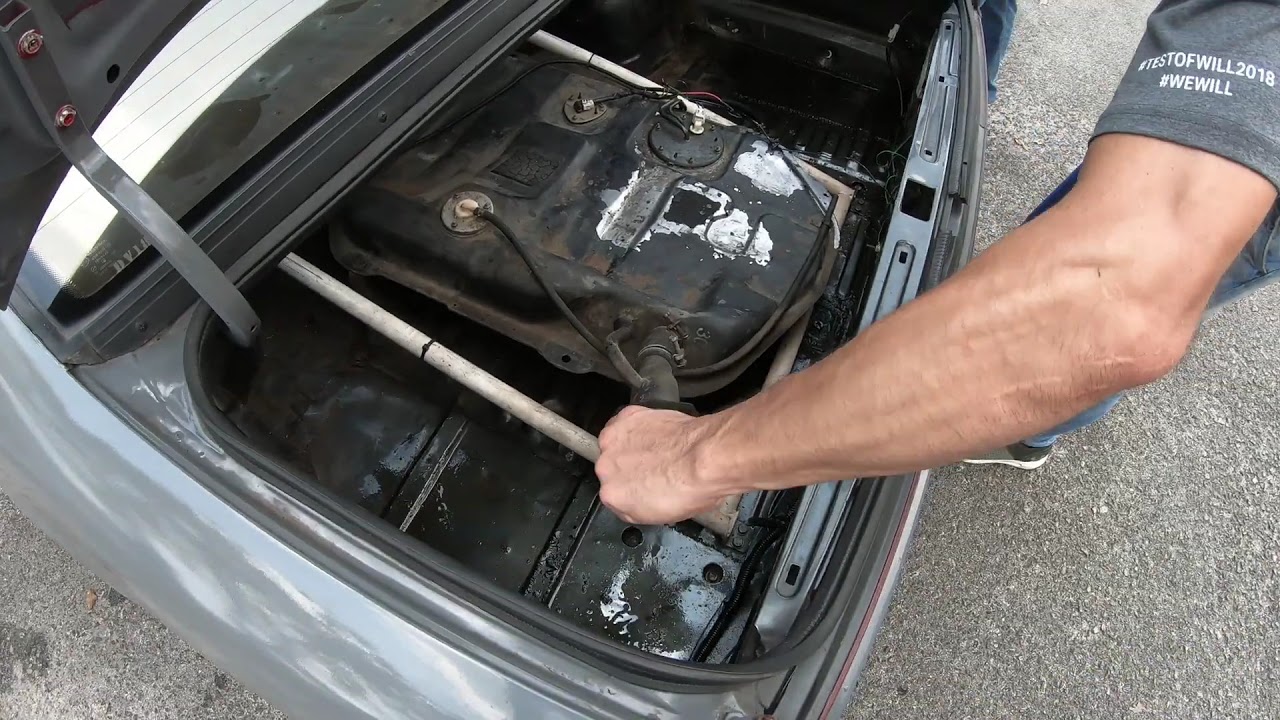This horizontal rectangular picture captures a man working under the raised hood of a gray or silver car. The engine compartment is somewhat grimy, with black metallic parts and patches of white powder or dried liquid scattered across it, contributing to a rusty appearance. Two wires extend from the engine, a black one and a partially red one, possibly connected to the battery or another part. The man's arm, adorned with visible hairs and veins, reaches down from the upper right corner, gripping something attached to the engine. He is wearing a gray short-sleeve t-shirt, with the sleeve bearing the inscription "Test of Will 2018, #WeWill." His blue jeans and gray shoes are partially visible. The action takes place on a rough, graveled outdoor surface, which is not smooth like concrete.